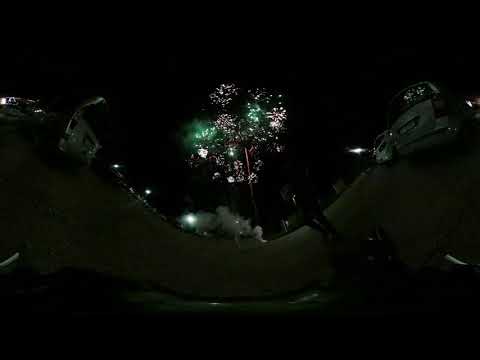The photograph captures an outdoor nighttime scene taken from inside a vehicle. The darkness of the night is punctuated by vibrant fireworks exploding in the sky, predominantly in green and purple hues, with some white accents. Smoke from the fireworks mingles with the dark sky, adding a hazy effect. The image exhibits a lens effect creating a u-shaped curve, making the sides of the photo appear higher than the center. This curvature frames the scene, where parked cars are visible on both sides and a shadowy figure, possibly a man, is discernible walking across the scene. Additional details include scattered specks of light that are hard to identify and what seems to be a street lamp towards the left. The overall dimness and complexity of the image give it a surreal, almost space-like quality.